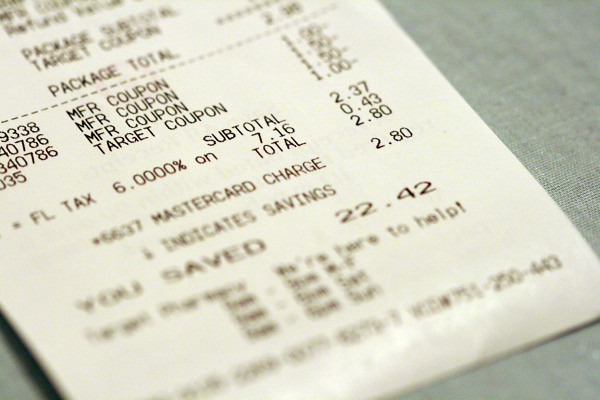A close-up image of the bottom section of a retail receipt, positioned at an angle, resting on a textured grey fabric. The fabric's texture is particularly noticeable on the right side adjacent to the receipt. The shot is tightly zoomed in, capturing intricate details of the fabric and the paper. The edges of the receipt at the top and bottom are blurred, directing focus toward the center. Prominently, the words "Manufacturer Coupon" and "Target Coupon" are printed three and four times respectively, and they are clearly visible. Detailed text including "Subtotal" and "Total" is sharp and legible as well. The receipt text also highlights, "You saved $22.42," emphasizing the customer's savings. The surrounding text, although slightly out of focus, remains decipherable, providing a comprehensive view of the receipt's detailed information.